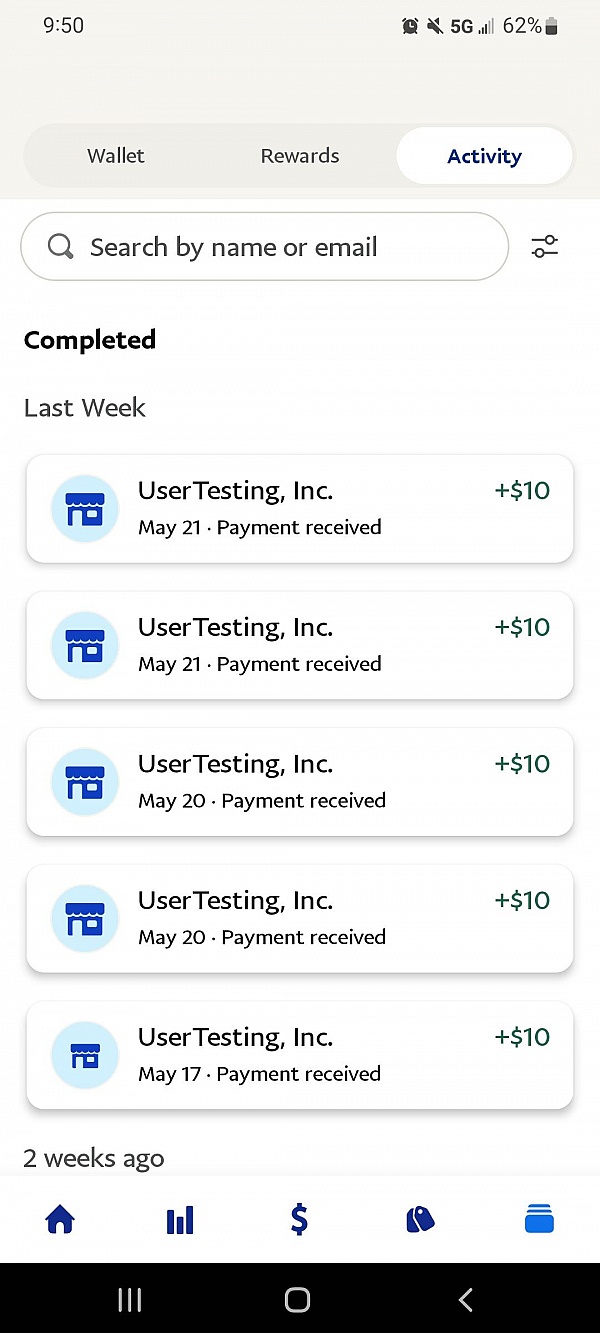This screenshot captures a detailed view of a user's activity on the mobile version of the UserTesting app. The top section features a dove-gray menu bar that reads "Wallet Rewards," with the "Activity" tab highlighted. A search bar invites users to "Search by name or email."

The activity section is organized under a header labeled "Completed" in bold text. Below, entries are categorized by time frames: "Last Week" and "Two Weeks Ago." Within the "Last Week" section, there are five entries, each detailing payments received from UserTesting, Inc.

- **Two payments** of **$10 each** were received on **May 21st**.
- **Two additional payments** of **$10 each** were received on **May 20th**.
- The earliest entry shows a **payment of $10** received on **May 17th**.

Each payment entry is accompanied by a distinctive icon resembling a light blue circle with a darker blue image, reminiscent of a storefront.

As the user navigates the app, the bottom menu provides various options symbolized by icons:

- A home screen icon
- Graph bars that likely represent usage data or earnings
- A dollar sign, possibly for cashing out or viewing total earnings
- Unidentified tags
- An icon depicting multiple screens

This comprehensive layout provides a clear overview of user activities, payment history, and navigational features within the UserTesting app.